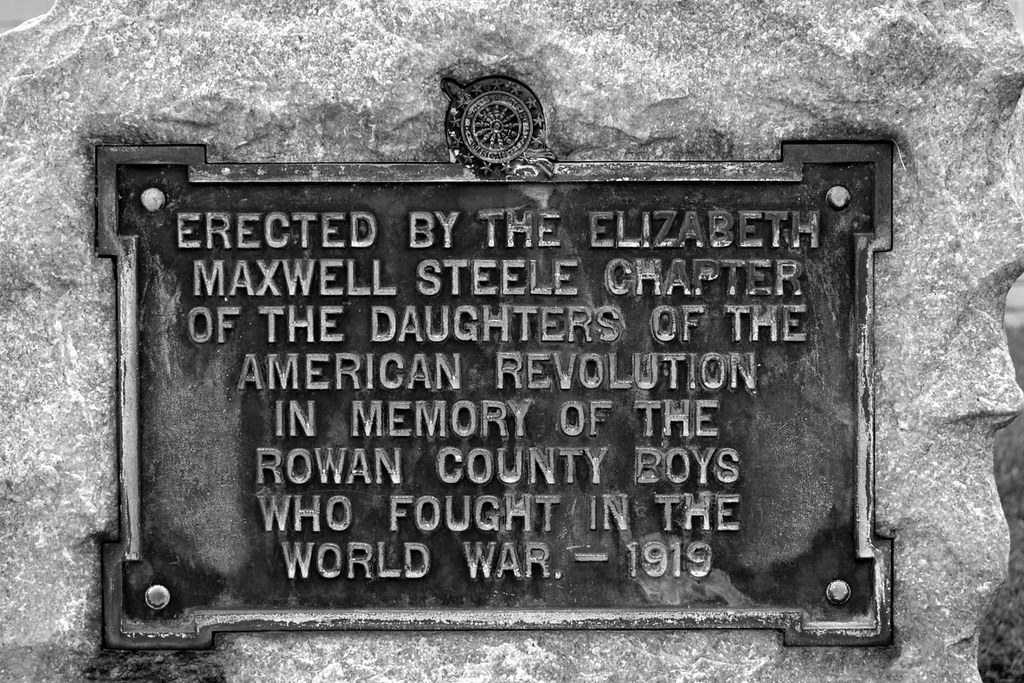This black and white photograph depicts a close-up view of a large, rough-textured gray stone wall with a metal plaque bolted at all four corners. The plaque appears to be made of a dark-colored stone, either black or gray, and is rectangular with slightly protruding squared corners. At the top center of the plaque is a circular emblem resembling a wagon wheel. The raised, capitalized text on the plaque reads: "Erected by the Elizabeth Maxwell Steele Chapter of the Daughters of the American Revolution in Memory of the Rowan County Boys Who Fought in the World War - 1919."